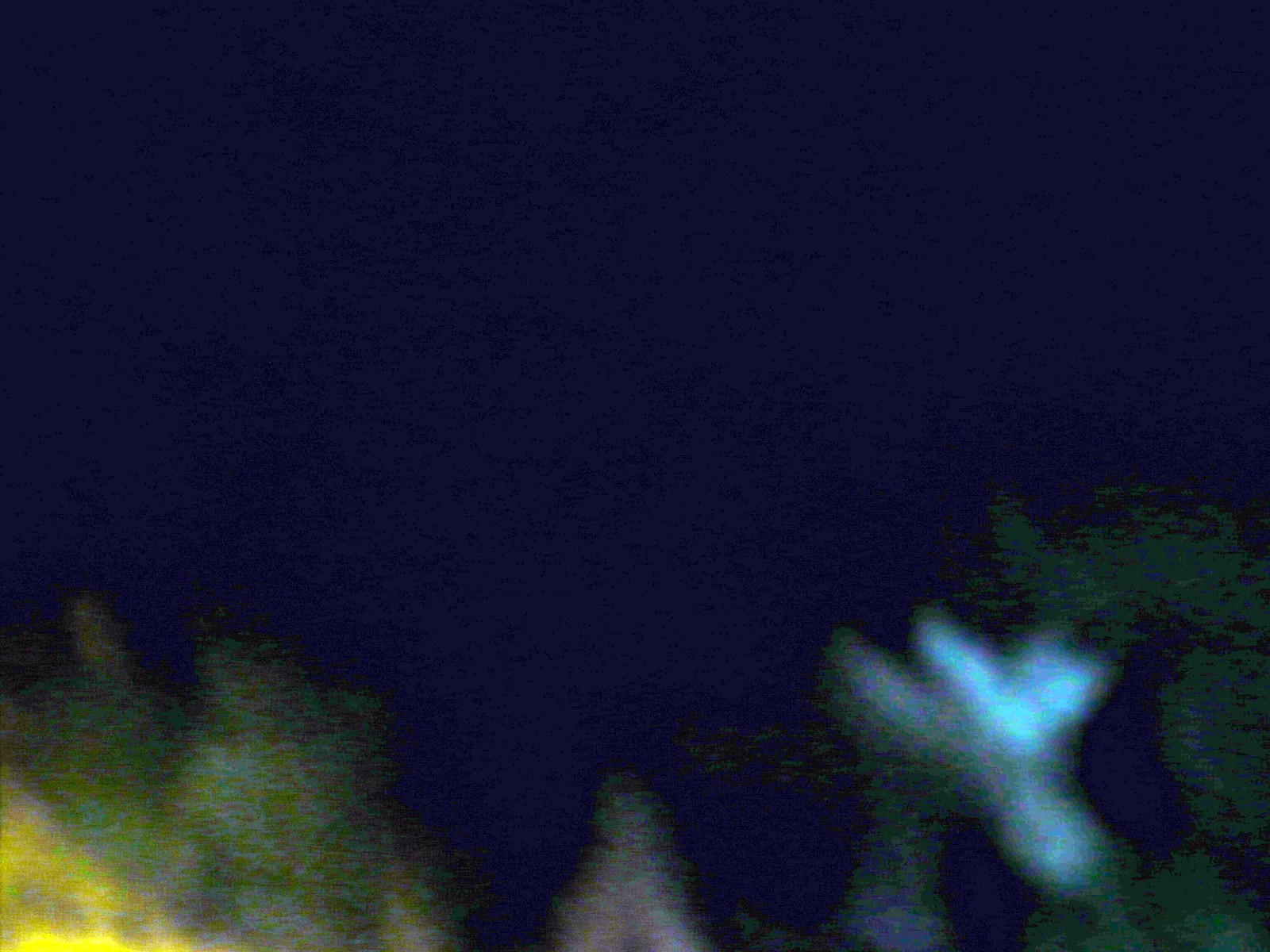The image is extremely blurry and appears to depict a landscape, possibly taken at night. The sky, which occupies the majority of the photograph, is a very dark navy blue. In the lower left corner, there's a small area, about an inch, of a yellow triangle glare. As we move towards the center bottom of the image, we see pixelated patches of green, likely representing the tops of trees. 

Centered at the bottom is a bright, blurry white shape that rises about an inch or two, resembling a mountain or perhaps a tree trunk. To the right of this white shape, there's more pixelated green, indicating foliage, and then a three-inch stretch of bright white continues along the bottom. The bottom right corner of the image features a dark, obscure shape that is difficult to identify but vaguely resembles either a branch or a hand. The entire image is characterized by its extreme blurriness and pixelation, making it difficult to distinguish precise details.